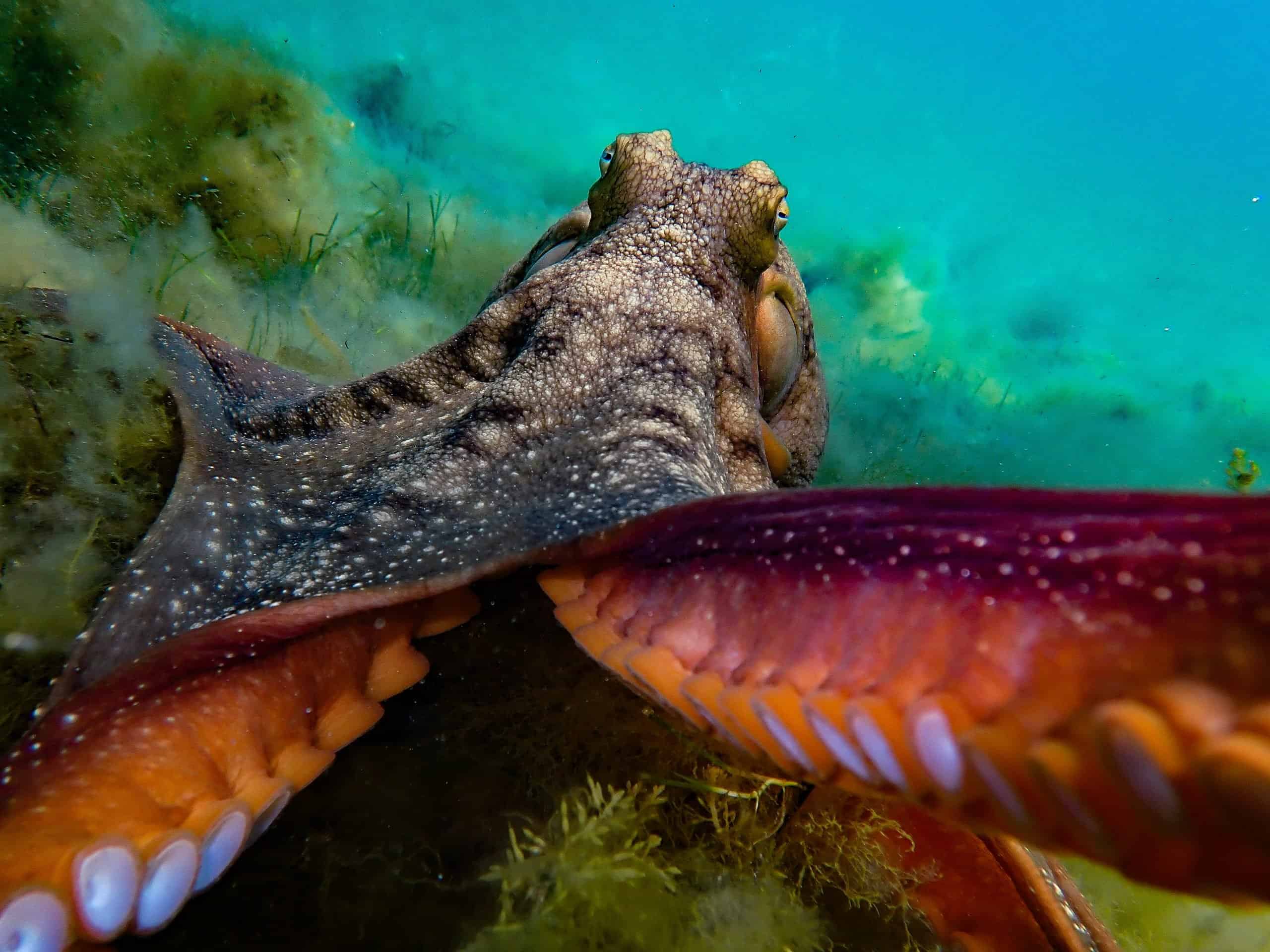This horizontally aligned rectangular underwater photograph captures the fascinating view of an octopus in its natural habitat. The background features the vibrant blue water with lush green seagrasses and seaweeds, adding richness to the scene. In the upper middle portion of the image, the octopus's head is visible, revealing its two prominent eyes that protrude frog-like from either side, adding a unique charm. The octopus displays a textured, bumpy skin that is grayish-brown with white speckles, merging into hints of yellow around the eyes. Centered and extending towards the bottom, its elongated tentacles reach outwards. The underside of the tentacles showcases a striking combination of maroon-red, orange, and yellow hues with pink undertones. The tentacles are adorned with white suction cups, each ringed with a yellow-orange outer coating. Beneath the octopus, additional green seaweed can be seen, providing a lush environment that highlights the creature's vivid coloration and intricate details.